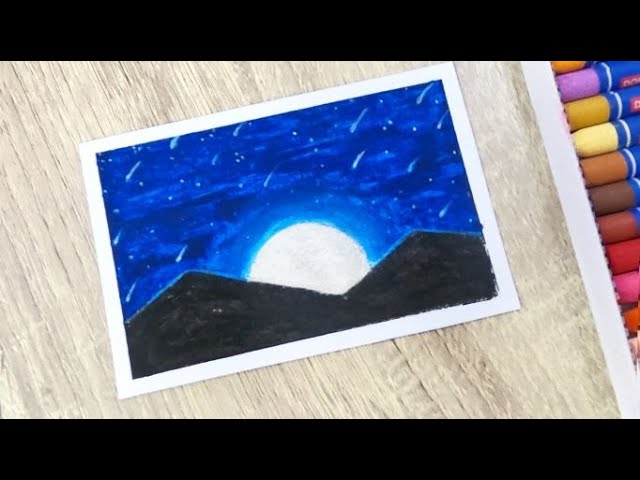The image is a stylized representation featuring a rectangular postcard set on a light grayish beige wood surface with vertical striations. The postcard, angled from right to left, depicts a serene night scene. At its top and bottom, black horizontal bands frame a minimalistic illustration of a white moon rising behind two black triangular hills under a star-studded gradient sky that transitions from dark blue to light blue. The entire scene is surrounded by a uniform white border, suggesting the postcard may have been created with pastels. To the right of the postcard, several colorful crayons are visible, hinting at the materials used for the artwork. The entire setup evokes a tranquil, almost otherworldly, desert landscape under the night sky.